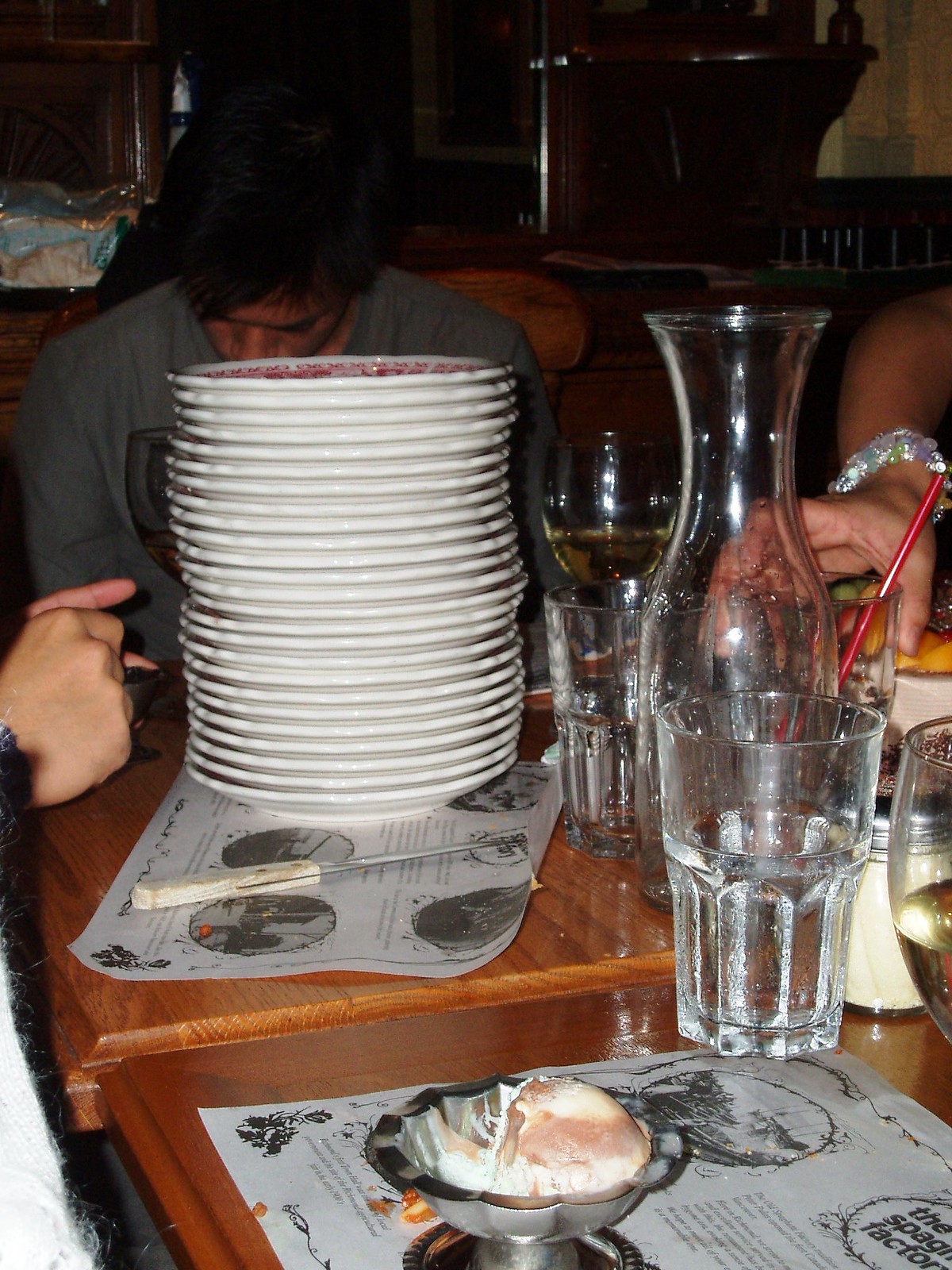In a dimly lit restaurant, the scene captures a man with shaggy black hair and long gray sleeves sitting at a brown table, looking down at his phone. He is partially obscured by a towering stack of approximately 20 white plates adorned with red patterns inside. This stack is centered on the table and sits atop a white piece of paper with illegible scribbles. A steak knife with a white handle rests on this paper as well.

On either side of the man, two other people are present, their arms partially visible. To the left, a clenched fist can be seen, while on the right, an arm bends downwards, reaching to grab a small glass with a straw. Surrounding the plates are various drinks, including a glass of water, a wine glass half-filled with Chardonnay, and a larger glass vase. The bottom foreground of the scene features a silver bowl containing half-eaten Neapolitan ice cream.

In the background, on the top left corner, a hint of a cabinet is visible, holding a blue dish with gold trim. Another brown cabinet is partially seen in the top right corner. The table is set with two placemats from the Old Spaghetti Factory, enhancing the restaurant's nostalgic ambiance.